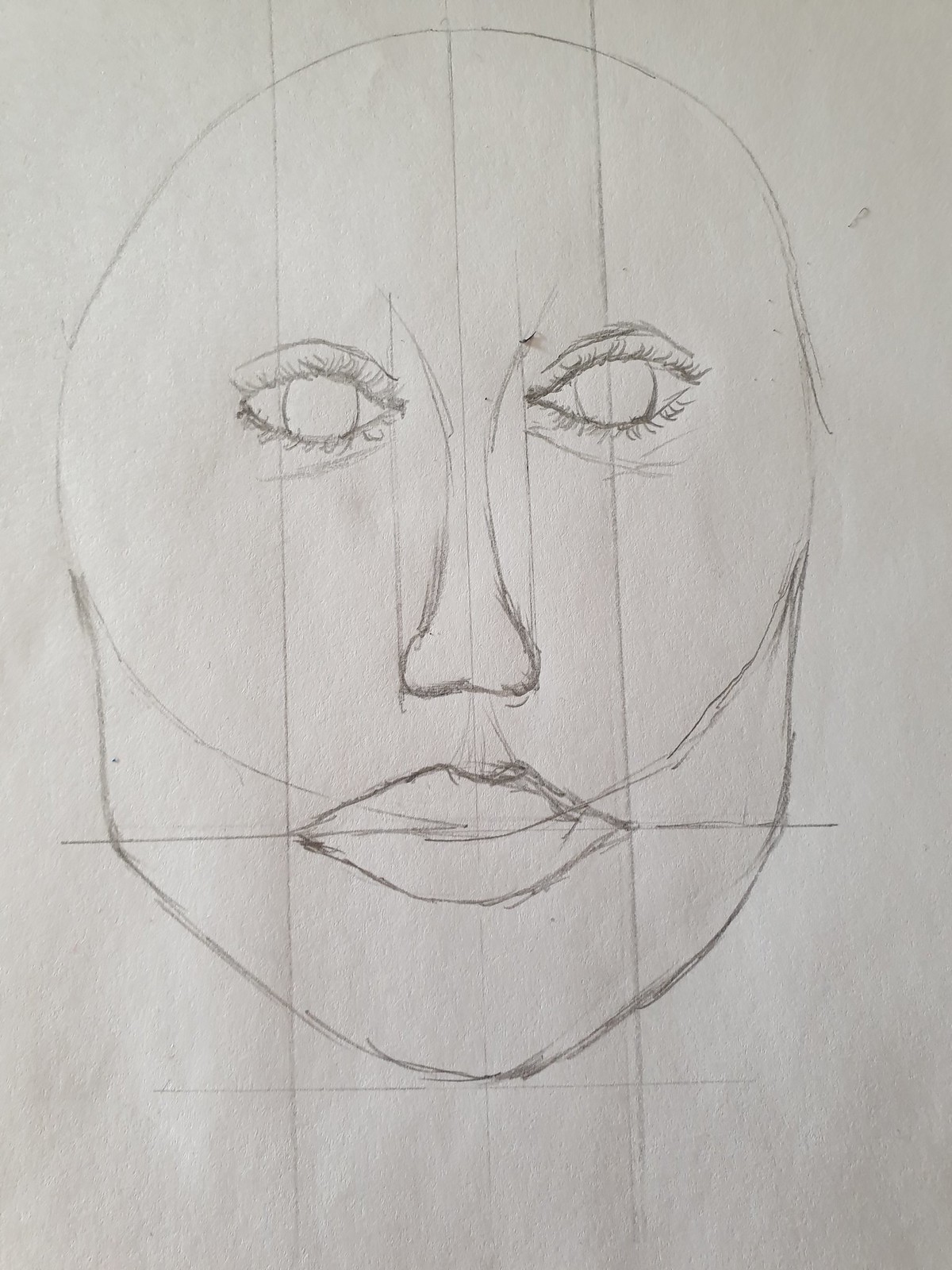A pencil sketch on a piece of paper captures the rudimentary outline of a human head. The drawing includes basic facial features: two eyes, a nose, a mouth, and a jawline that concludes in a defined chin. The image features multiple guiding lines, suggesting the artist was meticulously measuring to achieve proper facial proportions. The distance between the eyes appears to match the width of the nose, following classic drawing principles. Simple lines represent the eyebrows, while the eyes are depicted with large circles indicative of potential adjustment. The nose is outlined with straight lines extending from below the eyes, denoting its width. Similarly, the mouth’s position is calculated to align at a specific distance from the midpoint of the eyes. This sketch vividly illustrates the blend of preliminary rough outlines and the calculated efforts to determine facial proportions.